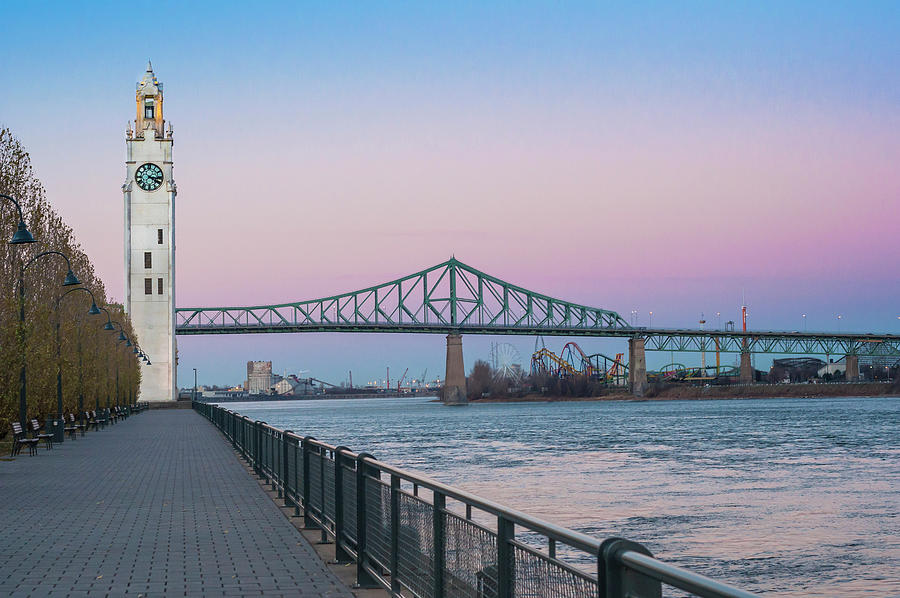This detailed image captures an outdoor scene at dusk with a striking combination of architectural and natural elements. To the left of the image, there's a well-maintained boardwalk lined with trees and streetlights, under which rows of benches sit. This walkway leads up to a tall, narrow, cream-colored clock tower with a blue clock face set to 3:20, and a cupola with a bell on top. Adjacent to the clock tower is a straight steel girder bridge that spans across a large body of water, extending from the right to the left of the image. The bridge appears to almost intersect with the clock tower but doesn't actually do so. In the background, under the bridge, a roller coaster's curved metal structure peeks through, adding a whimsical element to the scene. The sky, painted in hues of pink, blue, and white, indicates either sunrise or sunset, creating a serene and picturesque atmosphere. A metal fence along the water's edge ensures safety, while the calm water reflects the beautifully transitioning sky.